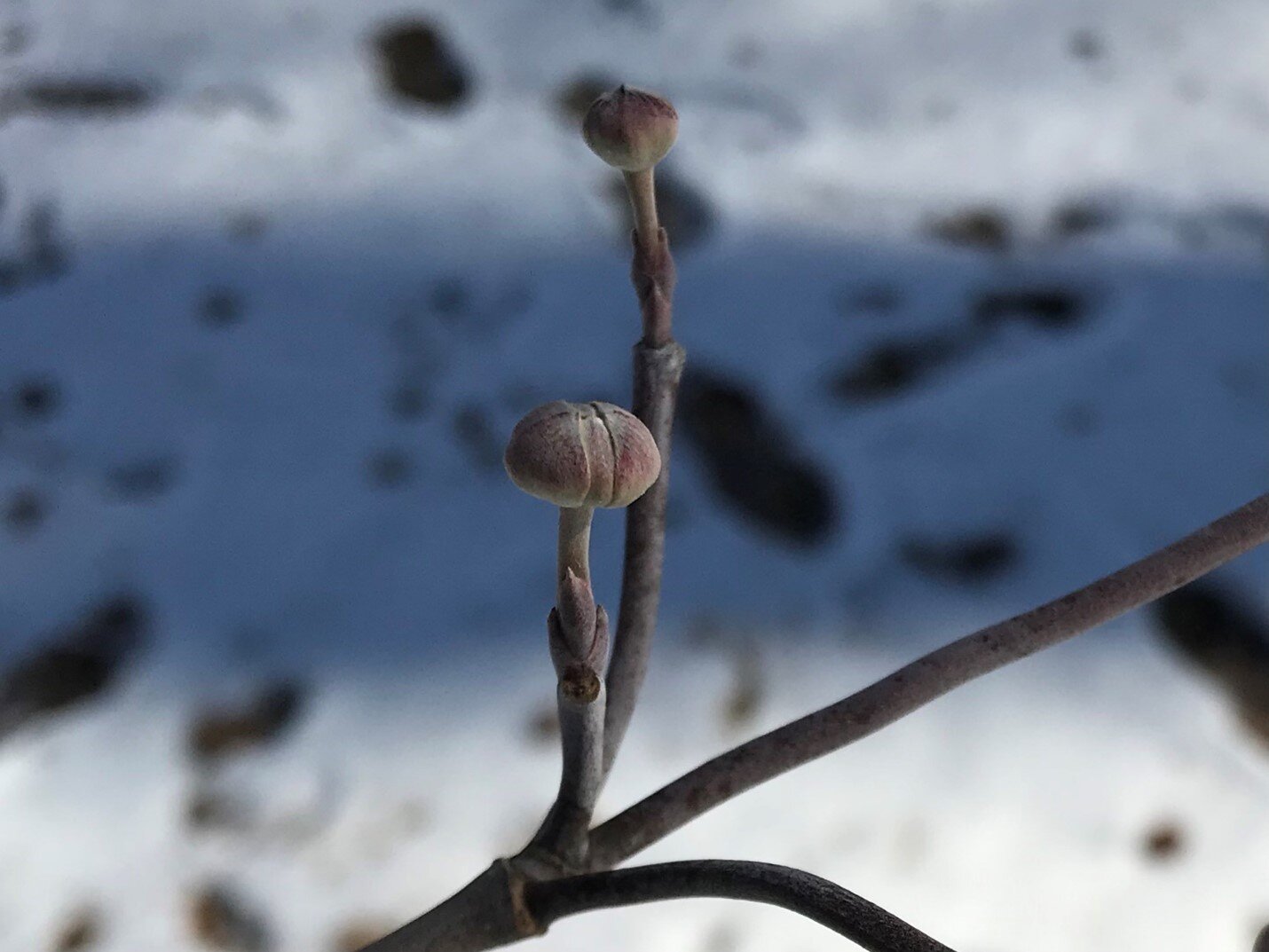This photograph captures a close-up view of a leafless plant branch during a winter scene, possibly transitioning to spring. The background is blurry, predominantly white, suggesting snow-covered ground, occasionally dotted with indistinct rocks, creating a fuzzy texture throughout. The lighting appears uneven with a large shadow cast across the ground, while sunlight peeks through, reflecting off the snow and illuminating the scene's top and bottom.

The main focus of the image is a dark gray branch or stem, shown in sharp relief against the hazy background. Two buds, poised to bloom, dominate this close-up. These buds have a dark purple hue, tinged with gray, likely due to the shadow they are partly under. One of the buds is positioned closer to the bottom left, while the other is slightly higher and more distant. The diagonal orientation of the branch adds a dynamic element, guiding the viewer’s eye upwards from the lower left to the middle right of the image.